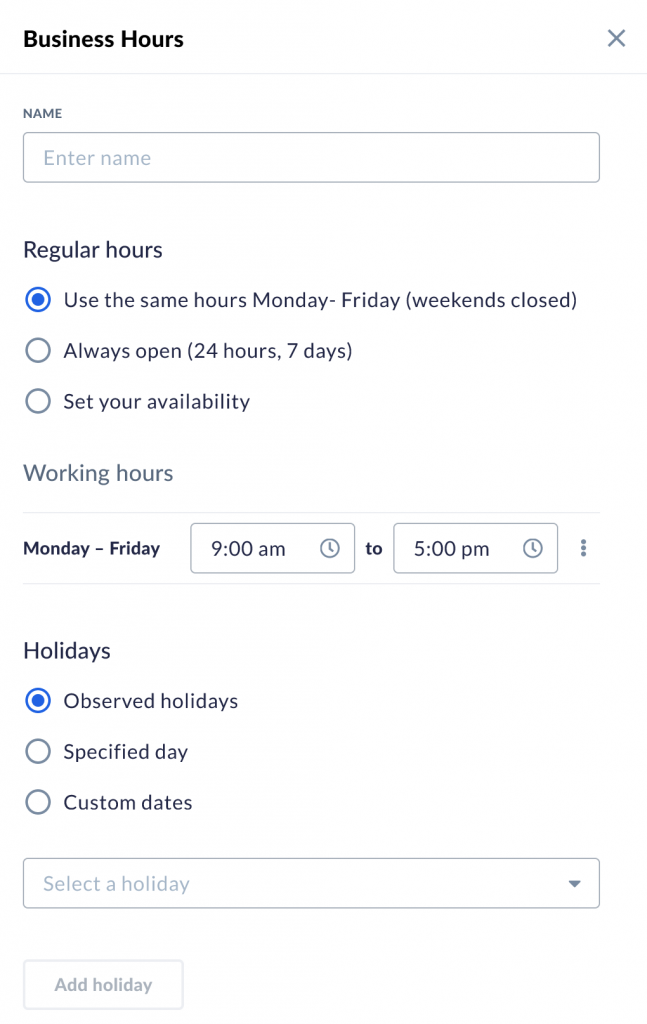The webpage features a clean, white background. At the top, the heading "Business Hours" is displayed in bold black text with an "X" icon to the right. A light gray line runs horizontally below the heading. 

Under this line, "NAME" appears in gray, capital letters above a text box labeled "Enter Name." Below that, is the heading "Regular Hours" in black text. Three radio button options are provided:
1. A selected option with a blue dot and background that reads "Use the same hours Monday through Friday" with the annotation "Weekends Closed."
2. "Always Open" with the annotation "24 hours 7 days."
3. "Set Your Availability."

The "Working Hours" section follows, featuring "Monday to Friday" with two input boxes displaying "9 a.m." and "5 p.m."

In the "Holidays" section, three additional radio buttons list different options:
1. "Observed Holidays," which is currently selected and indicated by a blue dot and outline.
2. "Specified Day."
3. "Custom Dates."

A drop-down menu beneath allows users to select a specific holiday, and a small rectangle below it labeled "Add Holiday" enables further customization.